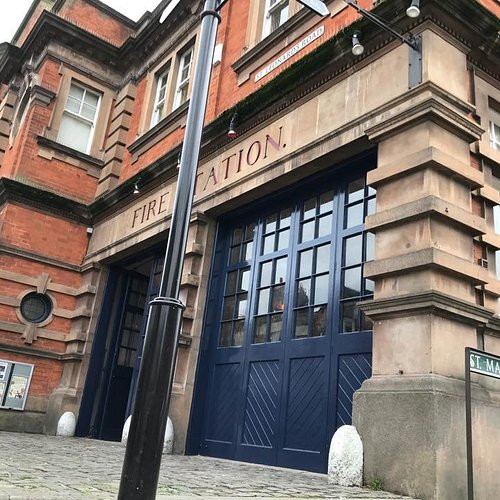The image showcases a detailed view of a modern fire station situated in an urban setting. The building features a prominent sign that reads "Fire Station," although the "S" is partially obscured by a black-colored metal pole extending upwards. The fire station wall is composed of gray wood, with vibrant orange (or possibly red) colored walls on the second floor. The architecture includes two very large entryways, one of which exposes a partially open blue garage door reflecting a building with a central light. Adjacent to the building, near the top right corner, a green street sign can be partially seen, reading "St. Ma," hinting at "St. Mary's" or "St. Mark's" Street, although the full name is not entirely visible. Additionally, a combination of colors such as blue, red, and yellow adorn the station, providing a cozy yet modern aesthetic. The structure is framed with white windows and possibly brick elements, while a pole structure and light post add to the unique visual elements.